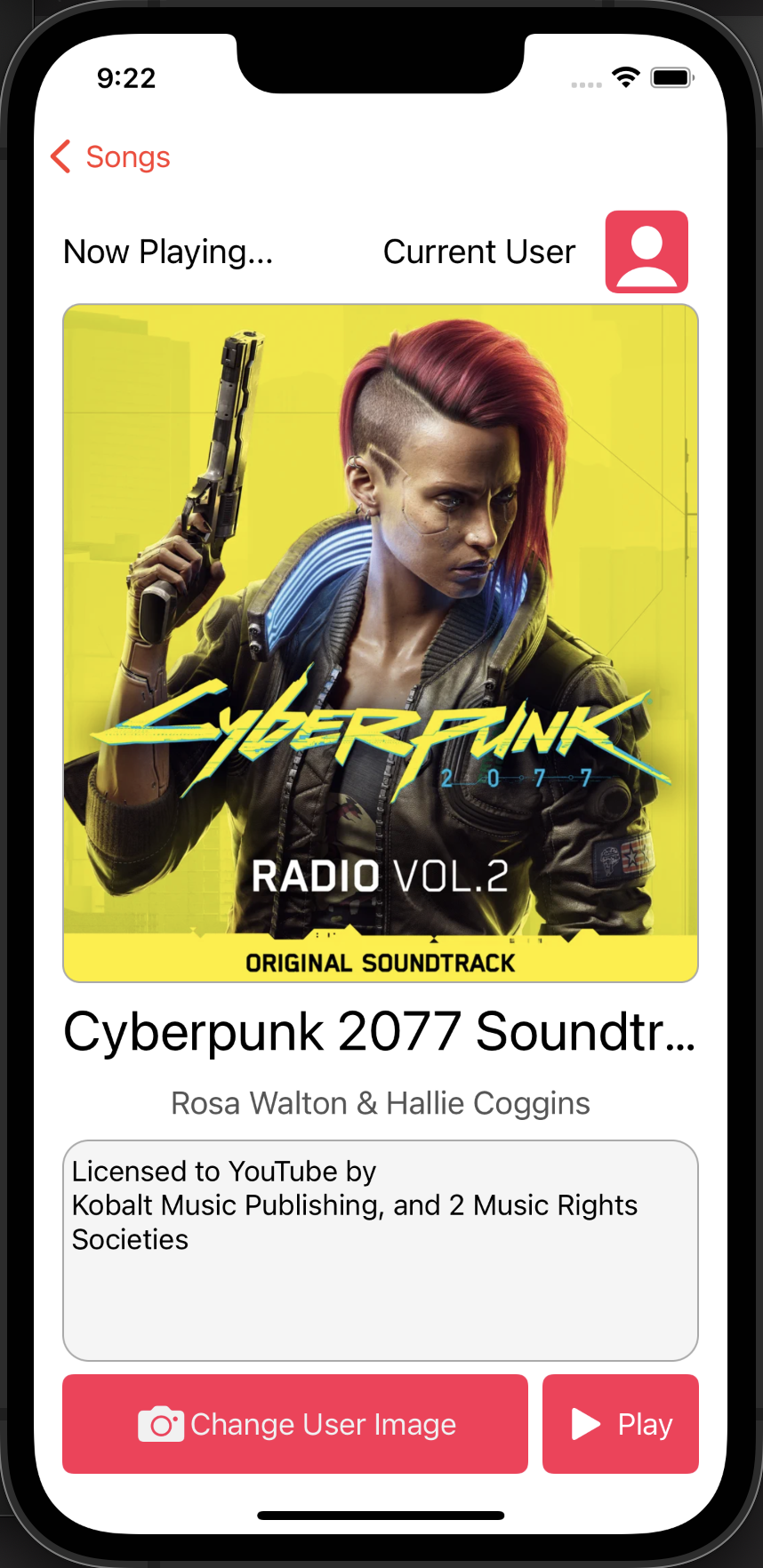The image features a cell phone screenshot encased in a black border on all sides. In the top-right corner, the time is displayed as 9:22, accompanied by an ellipsis icon, a full Wi-Fi signal, and a fully charged battery. On the top-left side, there is a red left-pointing arrow icon labeled "Songs," also in red.

Below this header, the text "Now Playing" is displayed, followed by "Current User" next to a generic profile picture. The profile icon has a red background with a white graphic representation of a head and shoulders.

Beneath this section, a yellow box contains an image of a woman with a partially shaved head, her remaining hair dyed fire-engine red and styled long on top. She is holding a pistol pointing upward and is dressed in a leather jacket. The text within this box reads, "Cyberpunk 2077 Radio Volume 2 Original Soundtrack."

Further down, the names "Rosa Walton" and "Hayley Coggins" are attributed to the music from "Cyberpunk 2077." At the bottom of the screenshot is a pink box labeled "Change User Name / Change User Image."